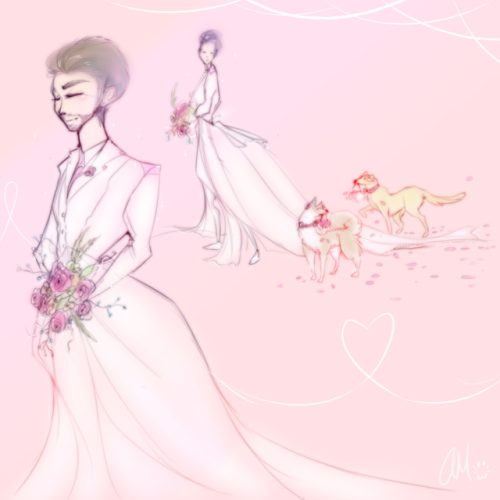The image is predominantly pink, with a pale pink background. In the foreground on the left side, there is a roughly outlined drawing of a person in a long, flowing dress that features long sleeves, a long train, and suit lapels, suggesting a combination of a traditional gown and a suit. This attire is pale pink in color and is paired with a shirt and tie underneath. The person, who has dark hair, heavy eyebrows, and facial stubble including a beard and mustache, is holding a bouquet of pink flowers and greenery.

Standing slightly behind this person is another figure, more indistinct but wearing a similar outfit with suit lapels and a long dress, also carrying a bouquet. Around these figures, two yellow dogs can be seen, one next to each person, adding a whimsical element to the scene. The dogs are holding bouquets or flower petals in their mouths.

The artwork exudes a delicate and soft quality, likely created with pencil or colored pencil, and showcases an intricate blend of bridal and groom elements in both characters, evoking a gentle and modern interpretation of traditional wedding attire.